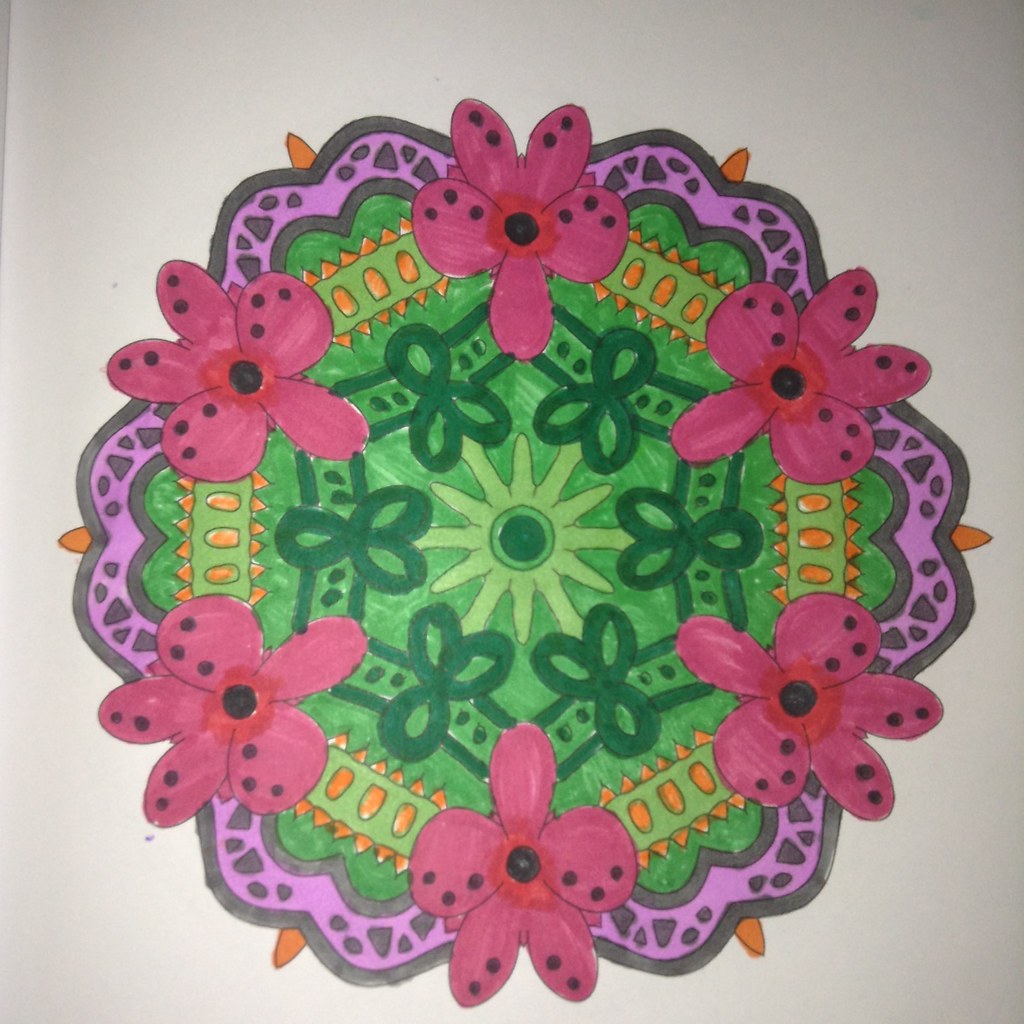This image showcases a meticulously detailed mandala drawing. Central to the intricate artwork is a hexagon with rounded sides, outlined twice and containing a unique formation of infinity symbols arranged symmetrically with two ovals at the bottom and one on top, connected by lines and filled with a sun-like design featuring a light yellow color, a green circle, and a black dot at the center. Surrounding this hexagon is a lumpy circular structure, primarily outlined in purple with a black border and filled with small black triangular shapes. Every two bumps of this periphery are adorned with vibrant pink flowers, each petal dotted in black except the central petal. Connecting these flowers is a continuous green stripe, accented with orange triangles along the outer edge and orange ovals within it. The interplay of colors and shapes creates a visually captivating and harmonious mandala.